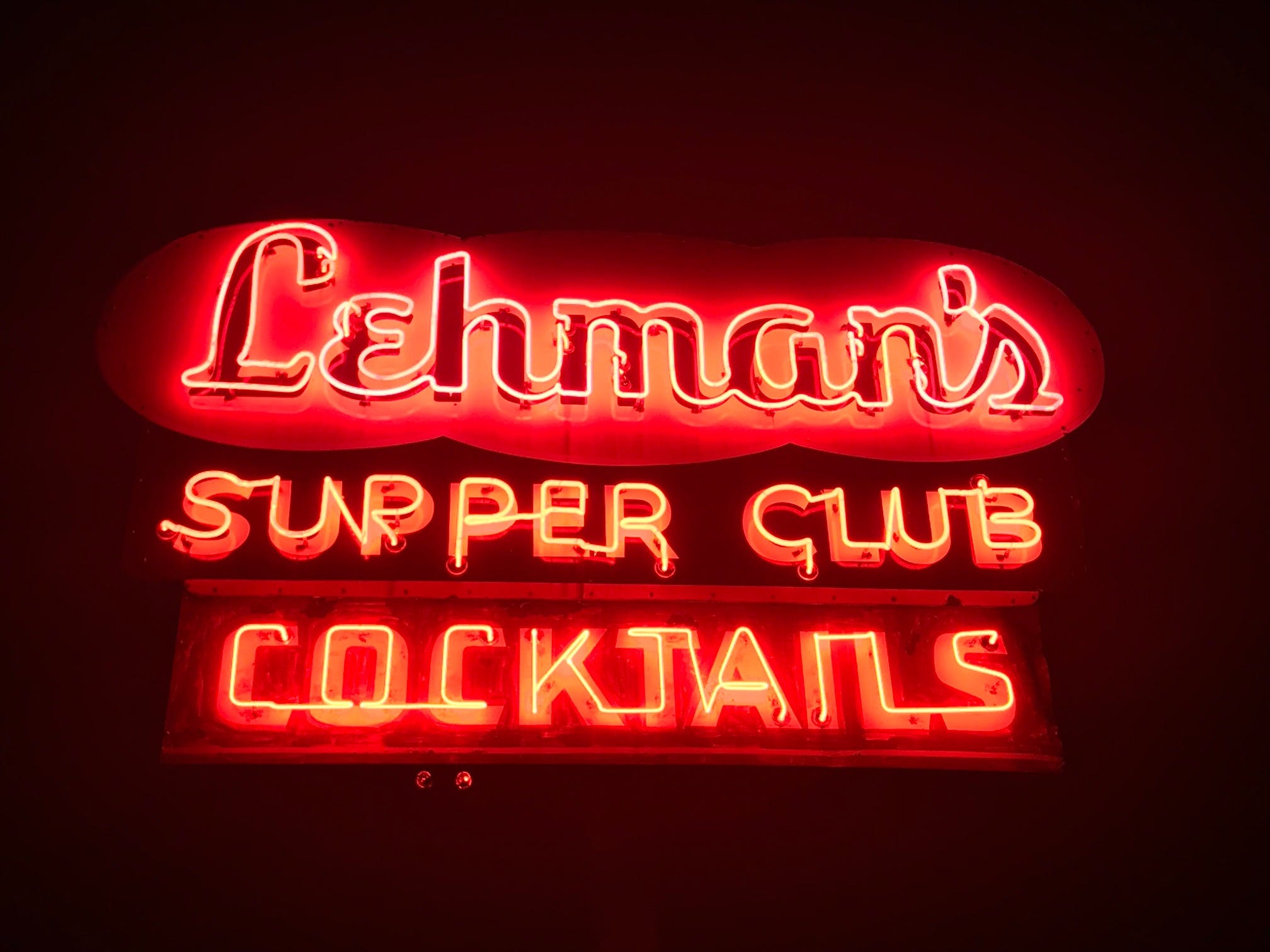This detailed photograph captures a professionally-taken, low-angle shot of a vibrant neon sign. The glowing sign prominently features the name "Lehman's" in illuminated white letters set against a fluffy oval background. Below, the term "Supper Club" is brightly lit in yellow against a red background, followed by a red rectangle displaying the word "Cocktails" in yellow neon lights. The color palette of the image consists of black, white, various shades of red, and orange, all contrasting against a dark, brownish-red to black background. This setup clearly signals the frontage of a restaurant or bar specializing in supper and cocktails. The composition and coloring of the sign emphasize its purpose and create a striking, visually appealing advertisement for Lehman’s Supper Club.